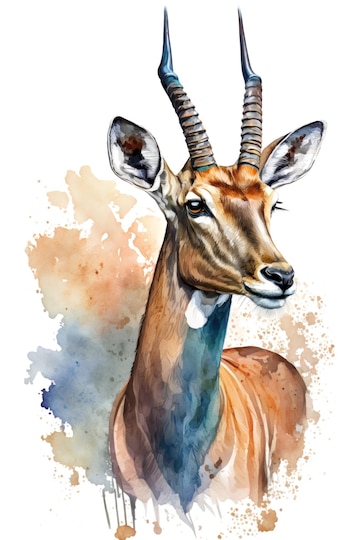This watercolor illustration features the head and upper body of an African antelope, likely a Springbok or gazelle. The animal, painted with meticulous care, has large ears that stick up attentively and straight, pointed antlers. The coloring predominantly consists of various shades of brown, with white accents around the mouth and under the neck. One noticeable eye is prominently displayed, capturing the animal's alertness. The neck showcases darker blue shadows, adding depth to the piece. The background fades into white, accentuating the detailed head and the upper body of the gazelle, rendered with both controlled and fluid brush strokes that evoke a sense of movement and liveliness. The watercolor technique gives a blend of sharp and soft textures, making the illustration vibrant and dynamic.